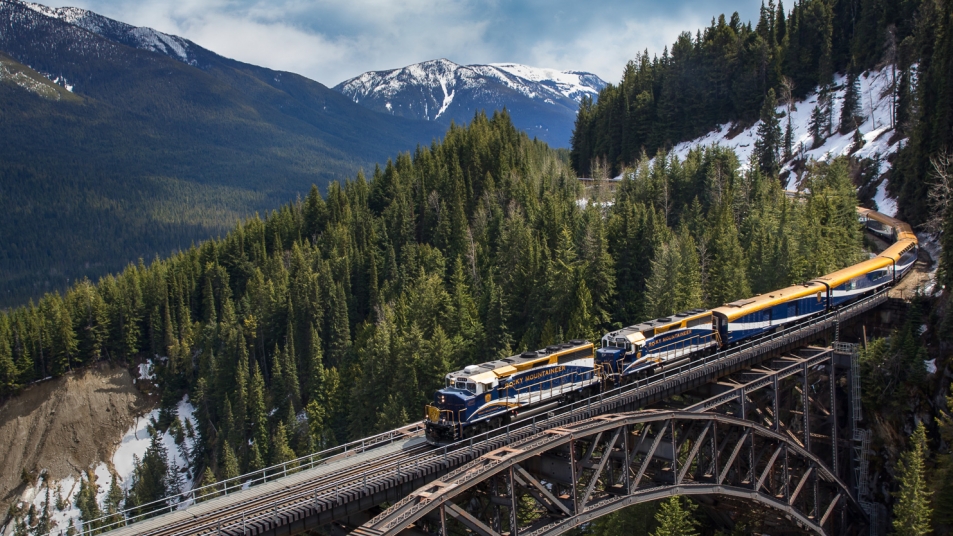The image depicts an outdoor, daytime scene showcasing a picturesque mountainous landscape intersected by a railway. Central to the image is a blue train with accents of yellow and white, positioned on a curved metal bridge that runs from the lower left to the middle right of the frame. The train, consisting of modern engines followed by passenger cars, travels along the trestle track that curves gracefully through the mountainous terrain. Beneath the bridge, the architectural metalwork spans a ravine, blending seamlessly into the natural environment.

The central portion of the image is dominated by a dense forest of tall green pine trees, beyond which lie majestic mountains. These mountains exhibit a vibrant mix of green at the base and snow-capped peaks, with the most prominent mountain occupying the left side of the image, gradually sloping from the bottom left to the upper right. Further in the distance, additional rugged mountain ranges rise, crowned with more snow.

Above this captivating landscape stretches a vast, azure sky dotted with large, white clouds, offering a striking contrast to the earthy and verdant tones below. The image overall exudes a serene yet dynamic ambiance, capturing the harmonious blend of human engineering and the breathtaking beauty of nature.